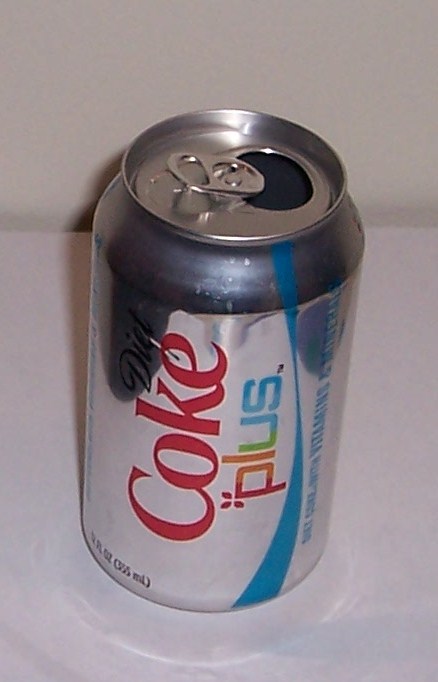This image showcases a close-up of an open can of Diet Coke Plus, prominently set against an off-white background on a white table. The can itself retains the classic silver shine distinctive of Diet Coke. The word "Coke" is displayed in red along the side of the can, with "diet" written in black above the "K" and "E". Below "Coke," the word "Plus" is written in a vibrant, multi-colored gradient: the "P" in red, the "L" in orange, the "U" transitioning from green on the left to blue on the right, and the "S" in blue. Enhancing its unique presentation, a blue ribbon design stretches vertically beneath the word "Plus," adding to the visual impact. There's also a mention of vitamins being added to this variant, suggesting a health-conscious twist to the drink. The can, noticeably opened with the tab lifted, reveals the metallic texture of the aluminum. The scene feels intimate and personal, likely a casual photo taken by someone rather than professional advertisement material, evoking a sense of pop-art reminiscent of Andy Warhol’s iconic work.